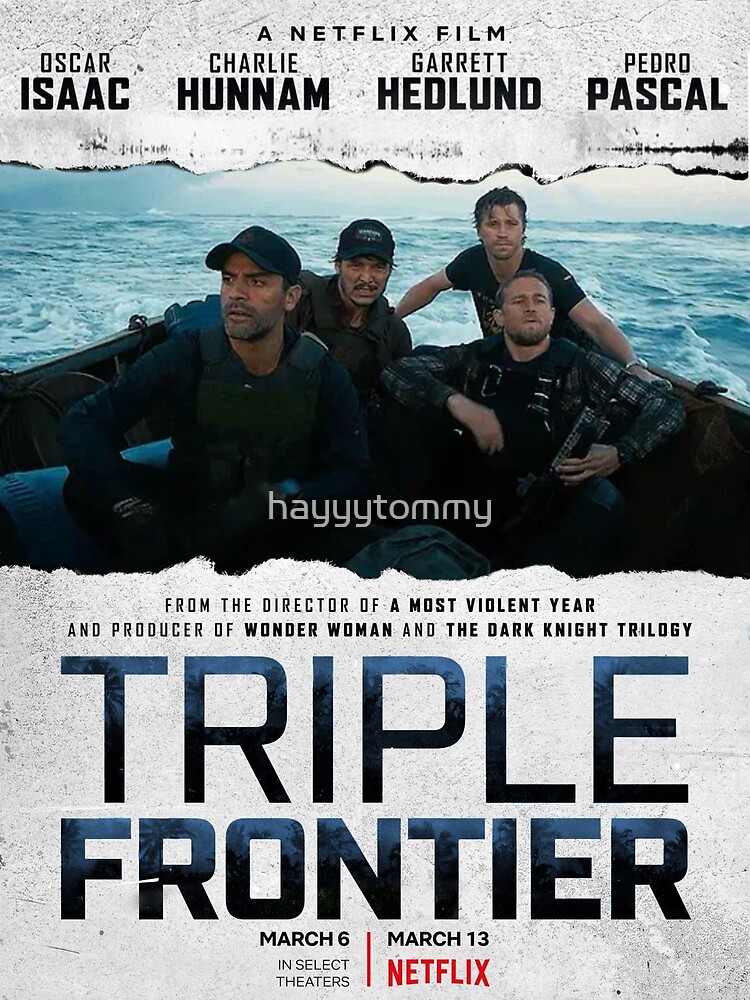This is a promotional movie poster for the Netflix film "Triple Frontier." The poster features a light gray background at the top and bottom, framing the central image. In the center, slightly towards the top, there is a dark photograph of four men in a small vessel or life raft floating on blue waters. The backdrop is a vast expanse of water meeting the sky. The men appear to be in military outfits, some wearing life jackets and others clad in black uniforms with black baseball caps. Notably, one man on the right is holding a rifle, and the man on the far left seems to be holding an indistinct item.

At the top center of the poster, in black lettering, it states, "A Netflix Film." The names of the leading actors are listed across the top: Oscar Isaac, Charlie Hunnam, Garrett Hedlund, and Pedro Pascal. Beneath their names and above the image, there is an intriguing line that reads, "Hey Tommy," stylized as "H-A-Y-Y-Y-T-O-M-M-Y."

Below the image, on the light gray background, the text highlights the creative team: "From the director of A Most Violent Year and producer of Wonder Woman and the Dark Knight Trilogy." The movie's title, "Triple Frontier," is prominently displayed in large, blue and black letters with a subtle overlay of trees. At the very bottom, the release dates are provided: "March 6th in select theaters" and "March 13th on Netflix."